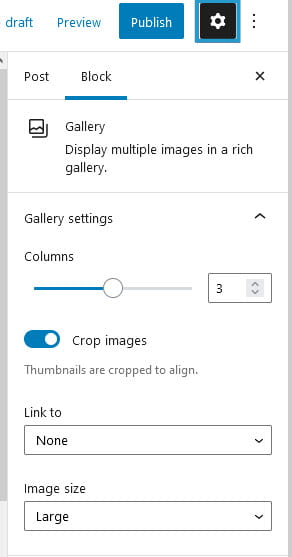The image captures a detailed view of a mobile interface, typically seen on an iPhone or Android screen, focusing on an application related to posting or editing content. Starting from the top, the screen showcases several options in lowercase blue letters such as "draft" and "preview" in an uppercase 'P,' positioned to the right. Following these, there is a navy blue square labeled "publish" in white letters, adjacent to another navy blue outlined square featuring a black square with a white star design in the center. To its right, three vertical black dots indicate additional options.

Below this row, the screen displays the phrase "post to" in black letters, situated to the right of a black X icon. A faint gray line follows, accompanied by a thicker, shorter blue line creating a division. Below this divider is another significant section: a box showing two square landscape icons stacked vertically, labeled "gallery" in black text to the right. Beneath this label, the text reads "Display multiple images in a rich gallery," followed by another faint gray line. Next, the term "gallery settings" appears, marked by an upward-pointing 'V' symbol.

Continuing down, the interface features a “columns” option with a slider bar positioned midway, marked by a circle that can be toggled. This slider separates a blue line from a gray one, next to a box displaying the number 3, indicating adjustments can be made. Below, there's a blue oval featuring a white circle pulled to the right, labeled "crop images" in black letters. Underneath, gray text explains, "thumbnails are cropped to align." The term "link to" is followed by a selection box reading "none," suggesting further options are available upon clicking.

Finally, "image size" is visible, followed by another selection box labeled "large." Two substantial gray lines flank this option on both sides, completing the interface layout.